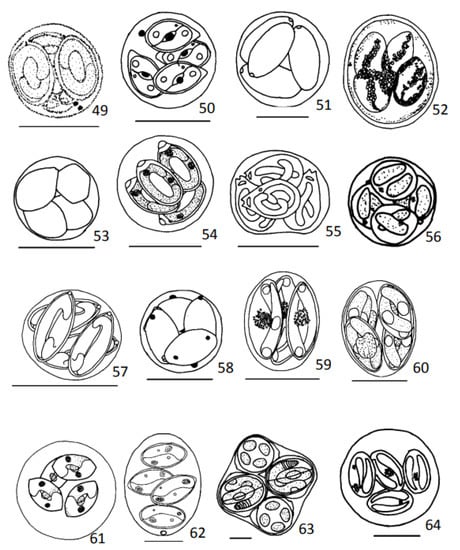This black and white illustration appears to be a scientific diagram rendered in pen and ink, resembling a set of meticulous microscope slides. The 16 round objects are arranged neatly into four rows and four columns, each labeled sequentially from numbers 49 to 64. The depiction primarily showcases various cell structures or microorganisms, potentially at different stages of embryonic development. Each object, contained within a small circle, exhibits unique internal configurations, suggesting detailed observation. Item number 55 notably resembles the shape of a fish, likely an incidental visual characteristic rather than an intended depiction. Despite some oblong or unconventional shapes, perhaps indicating cell division or differentiation, object number 63 distinguishes itself with a more rectangular form featuring rounded edges. This detailed illustration could serve as an educational tool, offering a visual reference for students or researchers in a classroom setting.